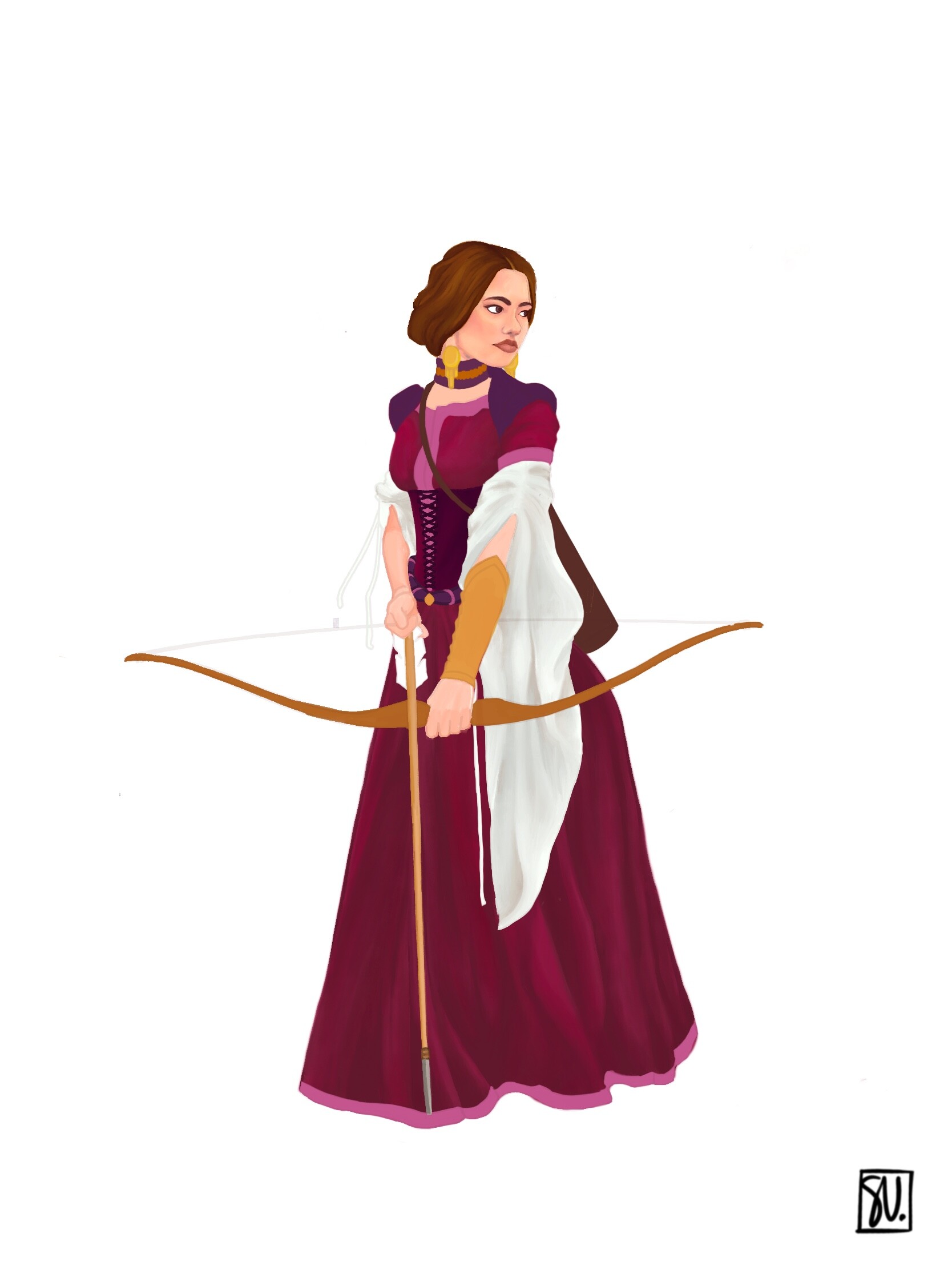The image showcases a hand-drawn illustration of a woman standing poised with a bow and arrow. She is dressed in a long, intricate magenta gown that flows from her neck to the ground, obscuring her feet. The dress features an array of details, including black epaulettes, a corset-like maroon bodice, and white sleeves that extend from her biceps to below her knees, contrasted against the rich magenta fabric. She wears additional protective gear on her left arm, designed for archery.

Her attire is further complemented by purple sleeves and a purple and gold choker adorning her neck. Golden earrings dangle from her ears, matching the choker's opulence. Long brown hair cascades down her back as she stands ready, gripping the bow in her left hand and the arrow's string in her right. The arrow points downward, yet she appears vigilant, looking intently to her left as though assessing a target in the distance.

The drawing is set against a white background, with a small black square in the bottom right corner enclosing the letters "A to U." The overall impression is one of steadfast readiness, capturing a moment of poised anticipation.